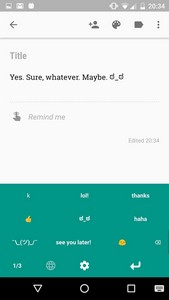The image depicts a screenshot of a website displayed on an iPhone. The top part of the screen is very blurry, shaded in gray, but some details are still visible. The battery life of the phone is less than half, and there is a strong connection signal. The time displayed appears to be 20:34, although the blurriness makes it somewhat unclear.

Beneath the status bar, there's a white navigation box featuring several icons. On the left, there is an arrow pointing to the left, followed by an icon of a person with a plus sign next to them. Next to that is an icon resembling a fan, and another box with an arrow pointing left. To the far right, there are three vertically aligned dots.

The website has a title that reads "yes sure whatever maybe," followed by some ambiguous text with "D_ D" and an underscore. The main body of the website includes a segment that says "remind me" next to an icon that looks like a fist with rays coming out of it. There is finely printed text mentioning "it is edited" and the date "2034."

At the bottom of the website is a green section filled with various icons and words. Some text reads "thanks haha see you later" with accompanying yellow icons of a thumbs up and a smiley face. Other elements include a star and a "K" in the upper left-hand corner. The bottom section of the screen displays the iPhone's typical navigation icons, including the home button and a square with an arrow, all in black.